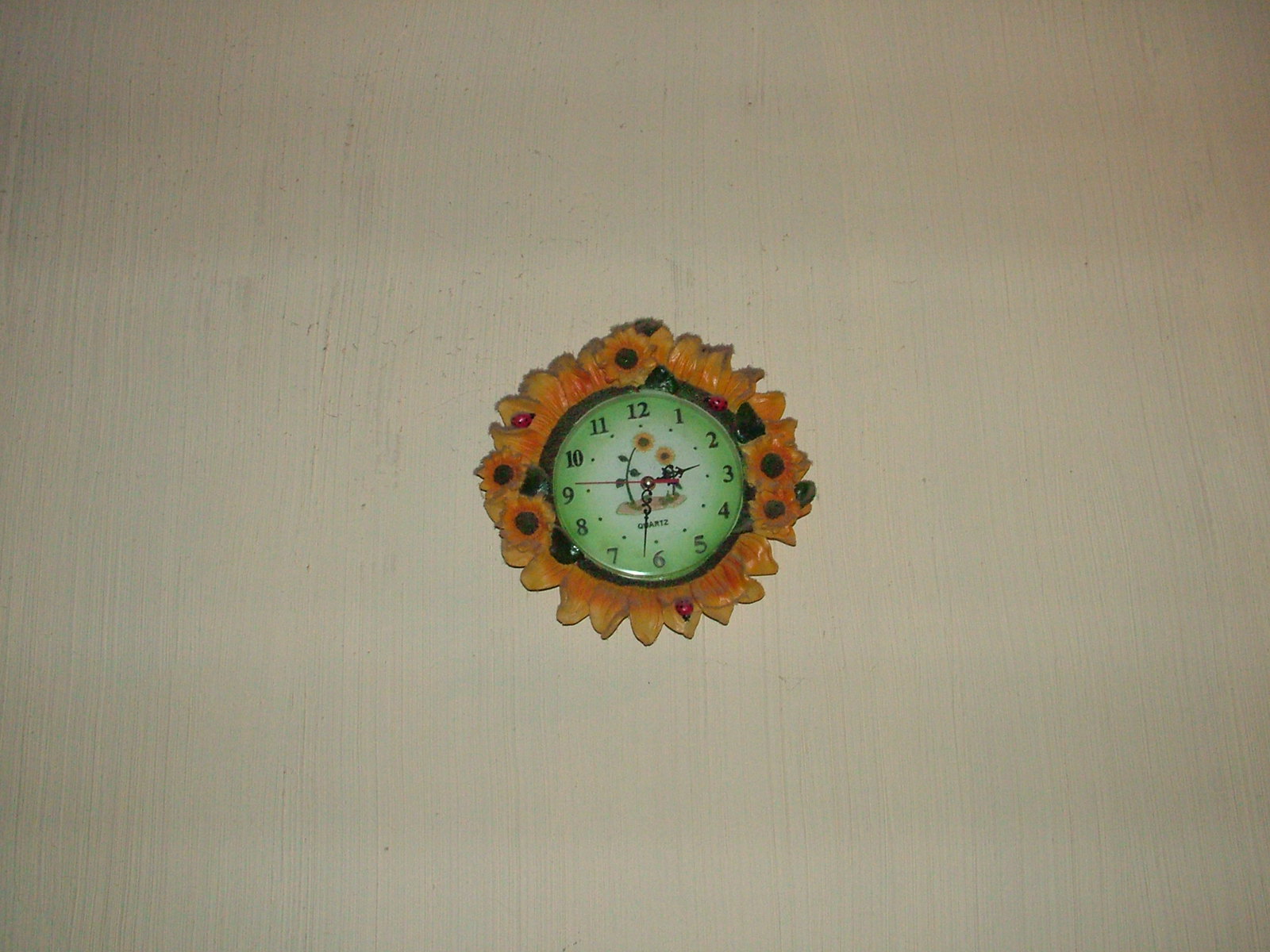The photograph features a predominantly white wall with a vertically grained texture, enhanced by a bright flash that highlights its uniform color. Centrally mounted on this wall is a small, decorative wall clock, taking up a relatively minor portion of the entire image—approximately one-tenth to one-fifteenth of the total space.

The focal point of the clock is its intricate design, resembling a sunflower. The face of the clock is green with black numbers around its perimeter, indicating hours 1 through 12. Surrounding this green face are vibrant yellow-orange petals, creating a vivid floral pattern. Additionally, at the 12, 3, and 9 o'clock positions, there are miniature sunflowers integrated into the design, adding a layer of intricate detail.

Inside the clock's face, beneath the ornate black hour and minute hands pointing to approximately 2:32, there is an illustration of two sunflowers growing from the soil, enhancing the botanical theme. There are also tiny red ladybugs located at the 6 and 10 o'clock positions, contributing to the clock's whimsical and antique charm. The clock's outer rim, slightly faded, consists of small ceramic sunflowers with subtle hints of red, evoking the feel of a cherished vintage piece.